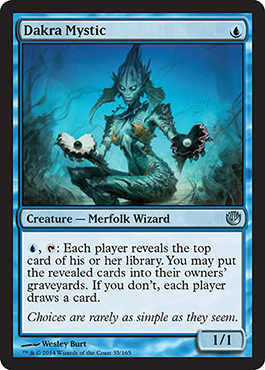A detailed caption for the image of the Magic: The Gathering card "Dakra Mystic" reads:

The image is a screenshot or scan of a Magic: The Gathering card, specifically the "Dakra Mystic" card. At the top, the card displays a blue rectangle bordered by a water-like motif, with the name "Dakra Mystic" written in black font. Below the name, there is a detailed illustration of the Dakra Mystic, a mythical merfolk wizard. The Dakra Mystic is depicted as a fish lady with human-like legs, seated on a rock underwater. She is holding open clams in both hands; the clam in her left hand contains a black pearl, while the one in her right hand holds a white pearl. Beneath the illustration, the card identifies the character as a "Creature - Merfolk Wizard" in black font. Further down, within a white rectangle, the card's ability is described: "Each player reveals the top card of his or her library. You may put this revealed card into their owner's graveyards, if you don't, each player draws a card." Below this descriptive text, in italics, a flavor text reads, "Choices are rarely as simple as they seem." Finally, the card's power and toughness are noted as "1/1" in the lower right corner.